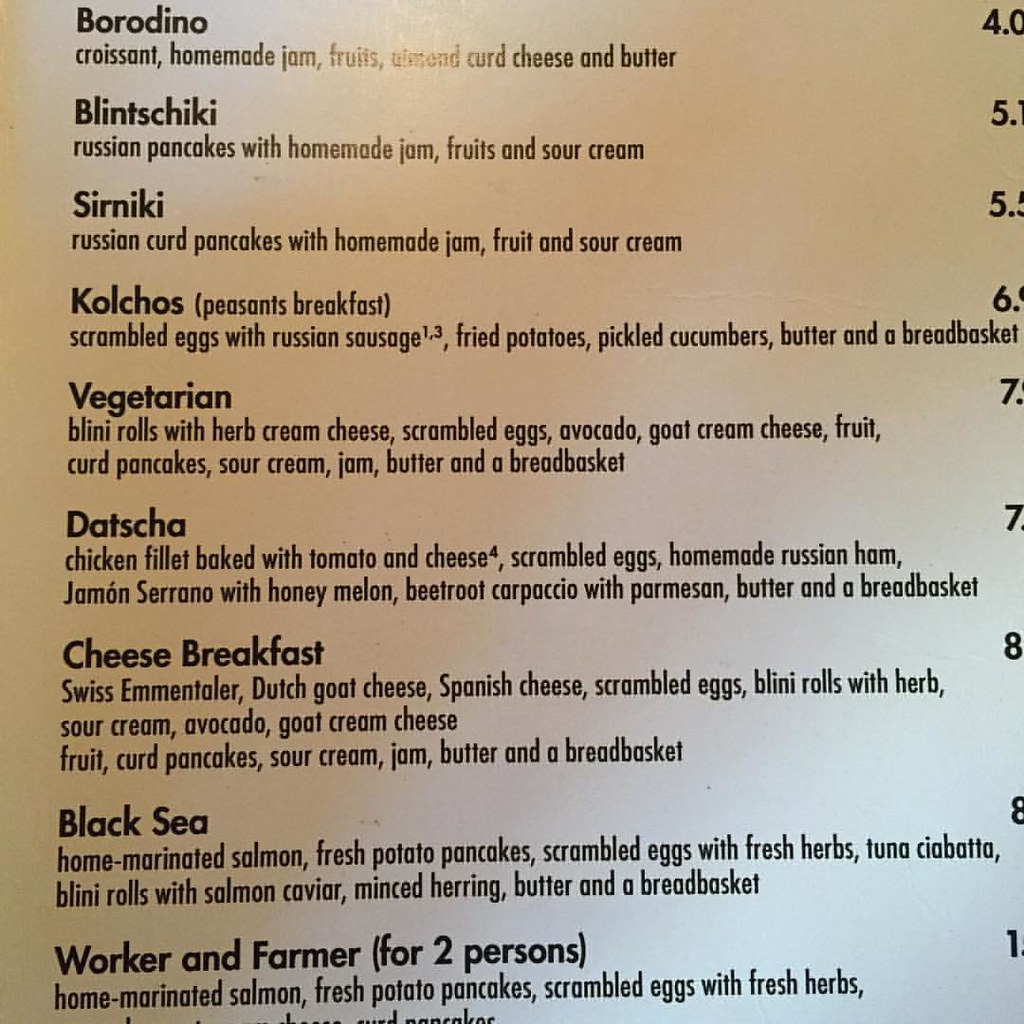The image depicts a detailed menu from a restaurant, prominently featuring various breakfast items along with their descriptions. At the top, the menu lists "Borodino," which includes a croissant, homemade jam, fruits, curd, cheese, and butter. Below that, "Blintschiki" is described as Russian pancakes served with homemade jam, fruits, and sour cream. Next, "Kolchoz" or the "Peasant's Breakfast" features scrambled eggs with Russian sausage, fried potatoes, pickled cucumbers, butter, and a bread basket. Following this is a vegetarian option comprising blini rolls with herb cream cheese, scrambled eggs, avocado, goat cream cheese, fruit curd, a pancake, and sour cream. Additional menu items include "Dacha," "Cheese Breakfast," "Black Sea," and "Worker and Farmer," the latter designed for two persons. The predominantly white menu displays both the dishes and their descriptions clearly, though most of the exact prices are partially cut off, showing only the main dollar amounts.